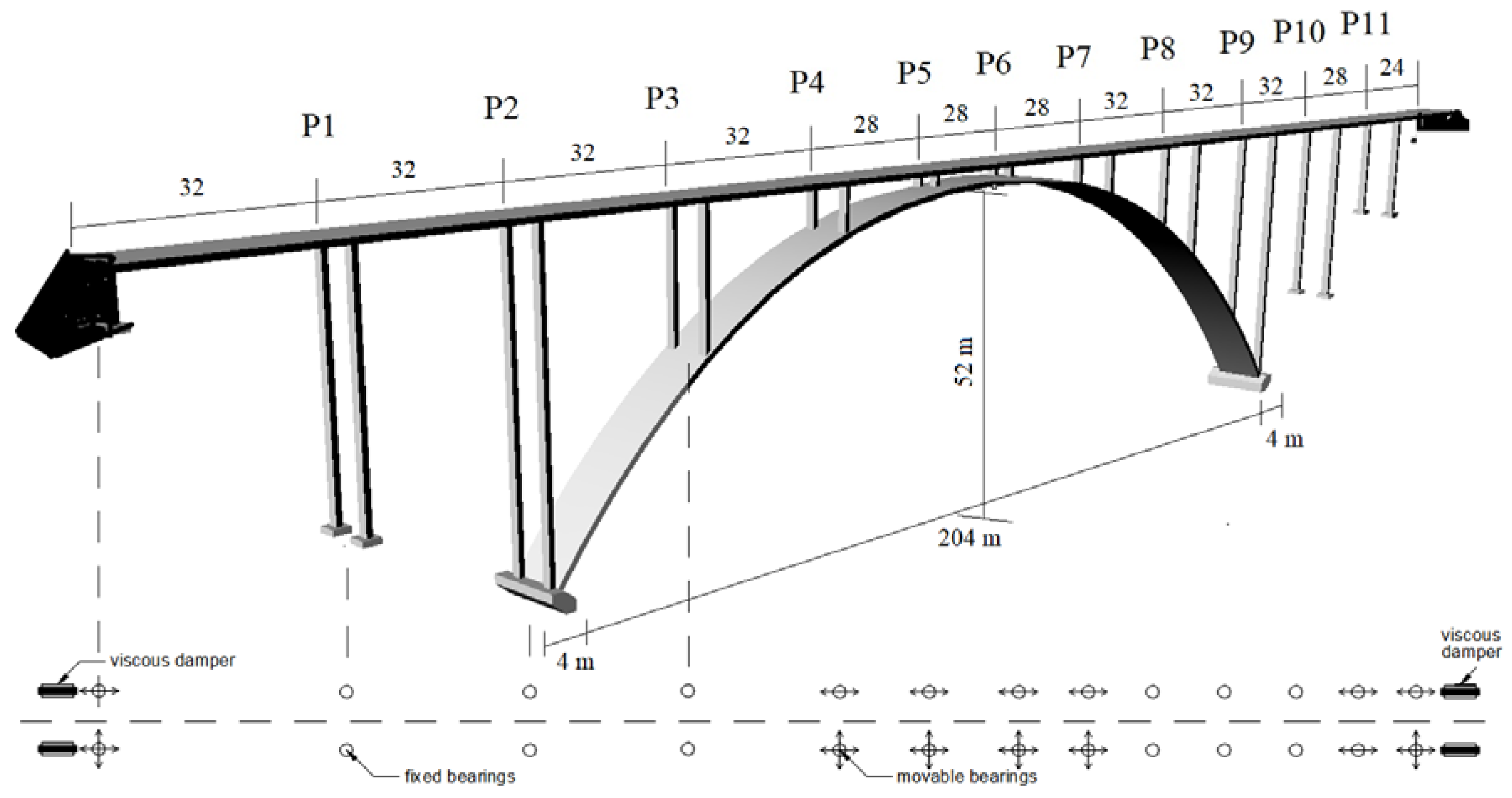The image is a detailed technical illustration of a bridge model, predominantly in black and gray, against a white background. The bridge spans horizontally from left to right with a slightly diagonal orientation and features a large curved arch underneath. The arch supports the bridge via a series of perpendicular posts. Each section of the bridge is marked incrementally from P1 to P11, indicating the attachment points to the arch below.

The dimensions of the arch are clearly noted, measuring 240 meters in length and 52 meters in height. Along the bottom of the image, various engineering components are labeled, including viscous dampers, fixed bearings, and movable bearings. These components are positioned at the bottom corners and along the base of the bridge. Additional measurements and annotations are dispersed throughout the illustration, providing further details about the bearings and structural elements.